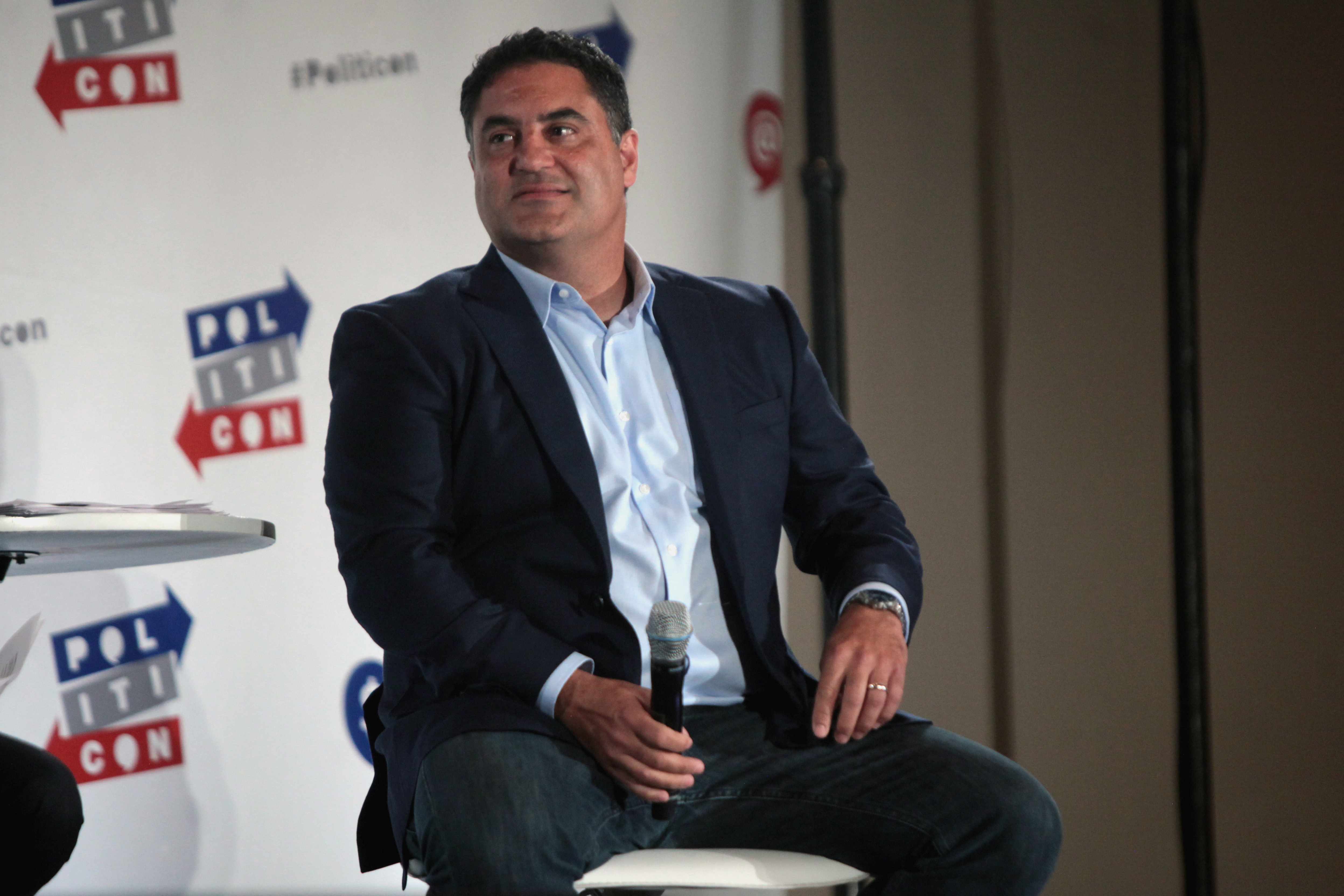The image captures a man seated in a white chair, likely from the political commentary show "The Young Turks." He has short black hair and a clean-shaven face, and he's dressed in a dark blue sport coat with a light blue button-down collared shirt. A gold wedding band adorns his left hand. The man is holding a black and silver microphone, appearing to be in the midst of an interview or discussion, as his head is turned to his right, looking off to the left side of the frame. Behind him is a notable white display banner featuring the Politicon logo in blue, gray, and red. The banner has blue arrows displaying "P-O-L," a gray rectangle with "I-T-I," and red arrows showing "C-O-N." To his left, there's a white table partially visible, and another individual is nearby, as suggested by a visible knee. The scene suggests a political event, reinforcing the professional and interview-like setting.